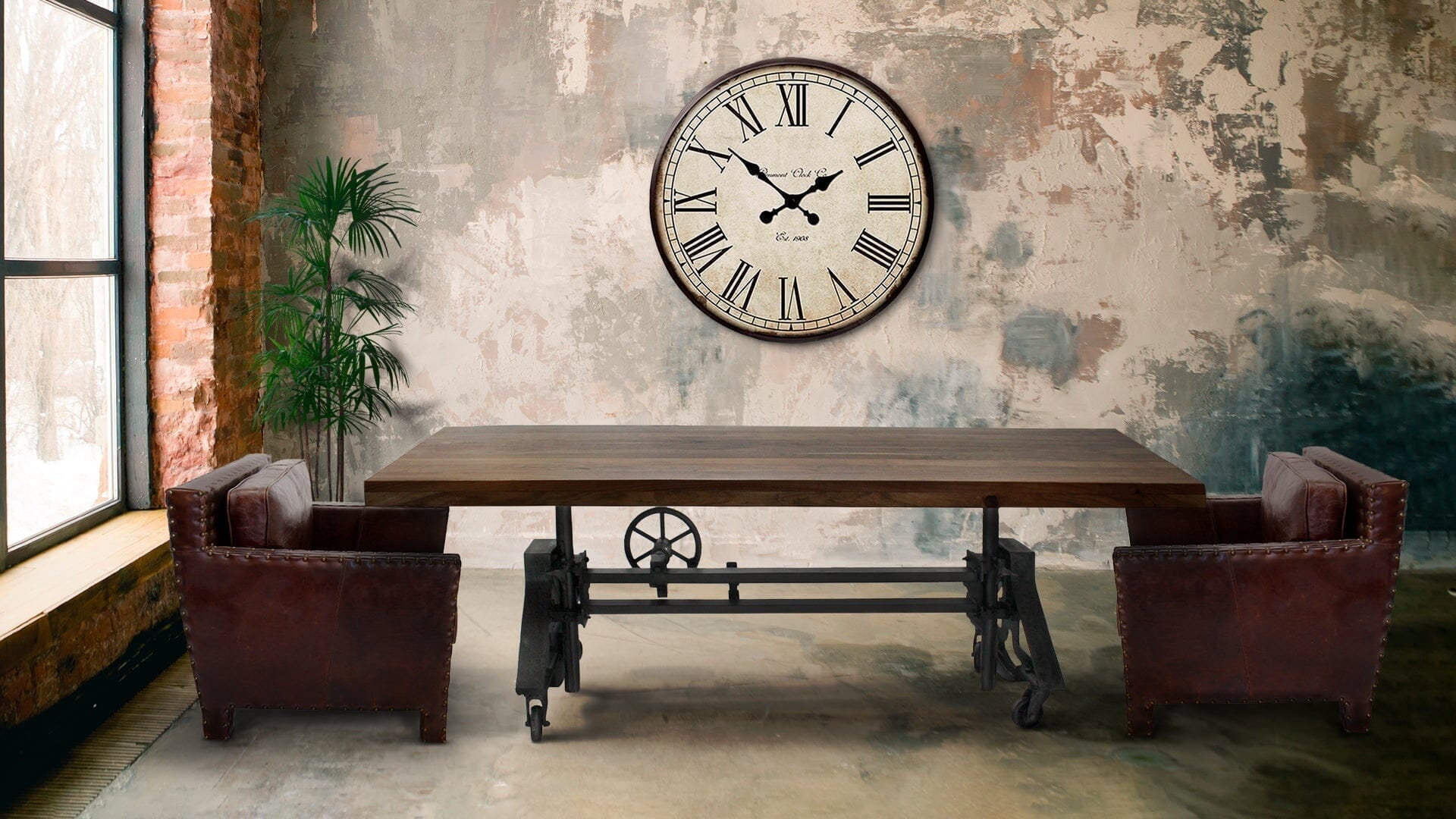The photograph captures a drab and dreary room, dominated by muted colors and an atmosphere suggesting neglect or abandonment. On the far left, a large window allows some natural light to seep in, contrasting with the overall dimness. Directly across from the viewer is a prominent clock featuring Roman numerals, mounted on a wall that appears to have a variety of faded colors, possibly achieved through a sponge painting technique.

Between the window and the clock, in the corner of the room, stands a tall potted plant with green, palm-like fronds, adding a touch of life to the otherwise lackluster space. The floor is bare cement, emphasizing the room's unfinished feel.

In the center of the room is a substantial wooden dining table with a retro-styled metal mechanism that suggests it can adjust in height. Flanking the table are two antiquated brown leather chairs, one on each end, embodying a blend of rustic and industrial design elements. The left side wall features exposed natural bricks, contributing to the room's eclectic and seemingly haphazard aesthetic.